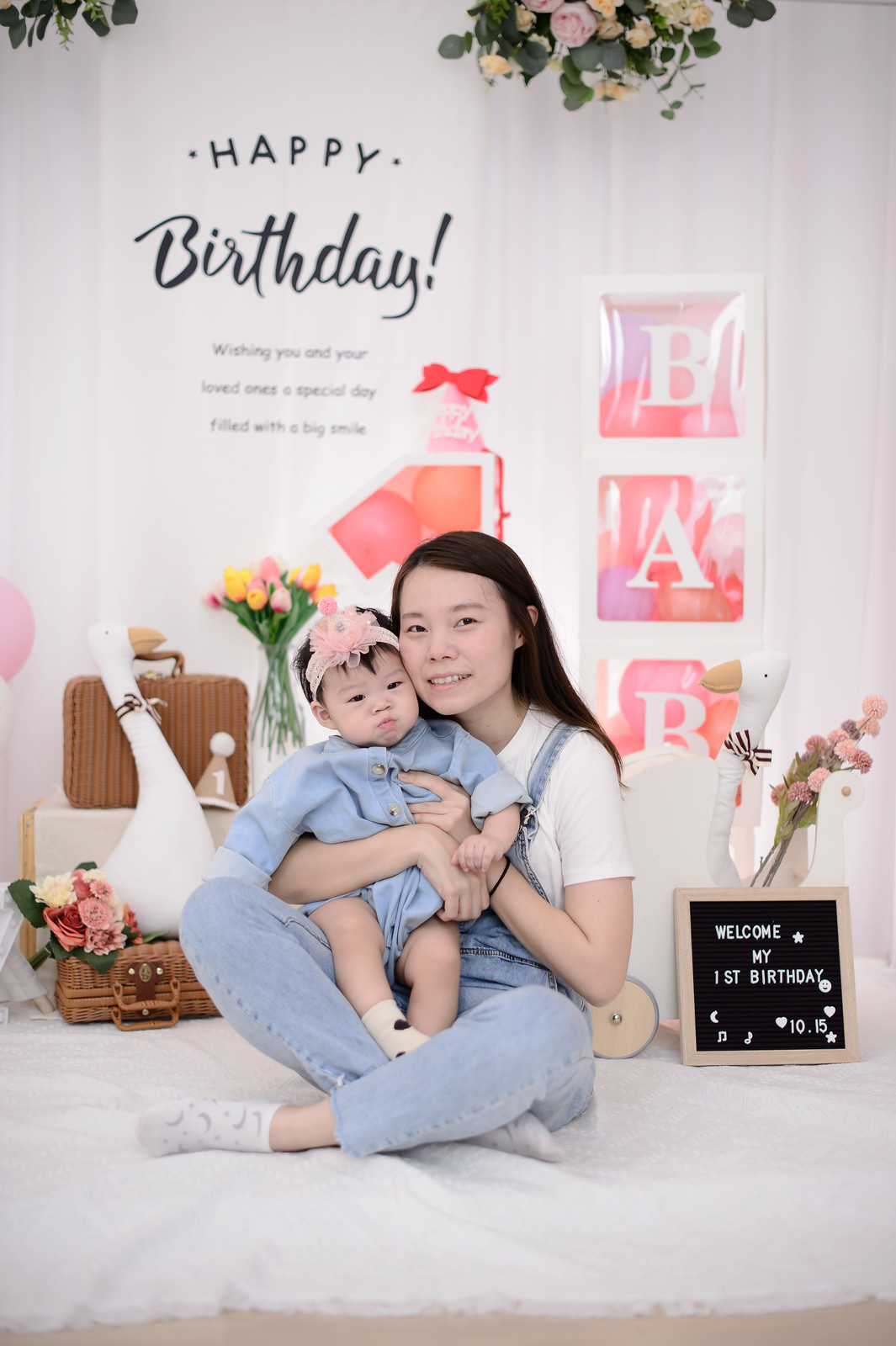The image captures a beautifully arranged birthday photo shoot in a studio, featuring an Asian young lady and a baby girl. The young lady, with long black hair, is seated on a mattress covered in white sheets. She is dressed casually in blue jeans, a jumper, a white t-shirt, and white socks. The baby girl on her lap is adorably dressed in a blue jeans dress and accessorized with a floral design hairband.

In the background, on the left side, there are small brown suitcases and bags, a bouquet, and a toy balloon shaped like a duck or crane. There is also a small birthday hat with the number one on it. The backdrop features a white decorative curtain with the text "Happy Birthday" in large, creative fonts. Below this, the message "Wishing you and your loved ones a special day filled with a big smile" is inscribed. Further down, there is an image of a flower bouquet.

On the top left and right sides of the curtain, flower decorations add to the festive ambiance. Directly behind the young lady’s head, the number one is prominently displayed with multicolored designs, a birthday cap, and a red ribbon. To the right of the lady, vertical blocks within the curtain spell out "BAB" in pink and purple balloon backgrounds, with the last block obscured by a white pillow and another crane toy. A small flower bouquet is positioned beside the blocks.

In the right corner, a wooden square-framed photo frame with a black internal area stands out. It bears the text "Welcome My First Birthday 10.15" along with stars, smileys, hearts, and musical notes in white fonts, completing the celebratory scene.